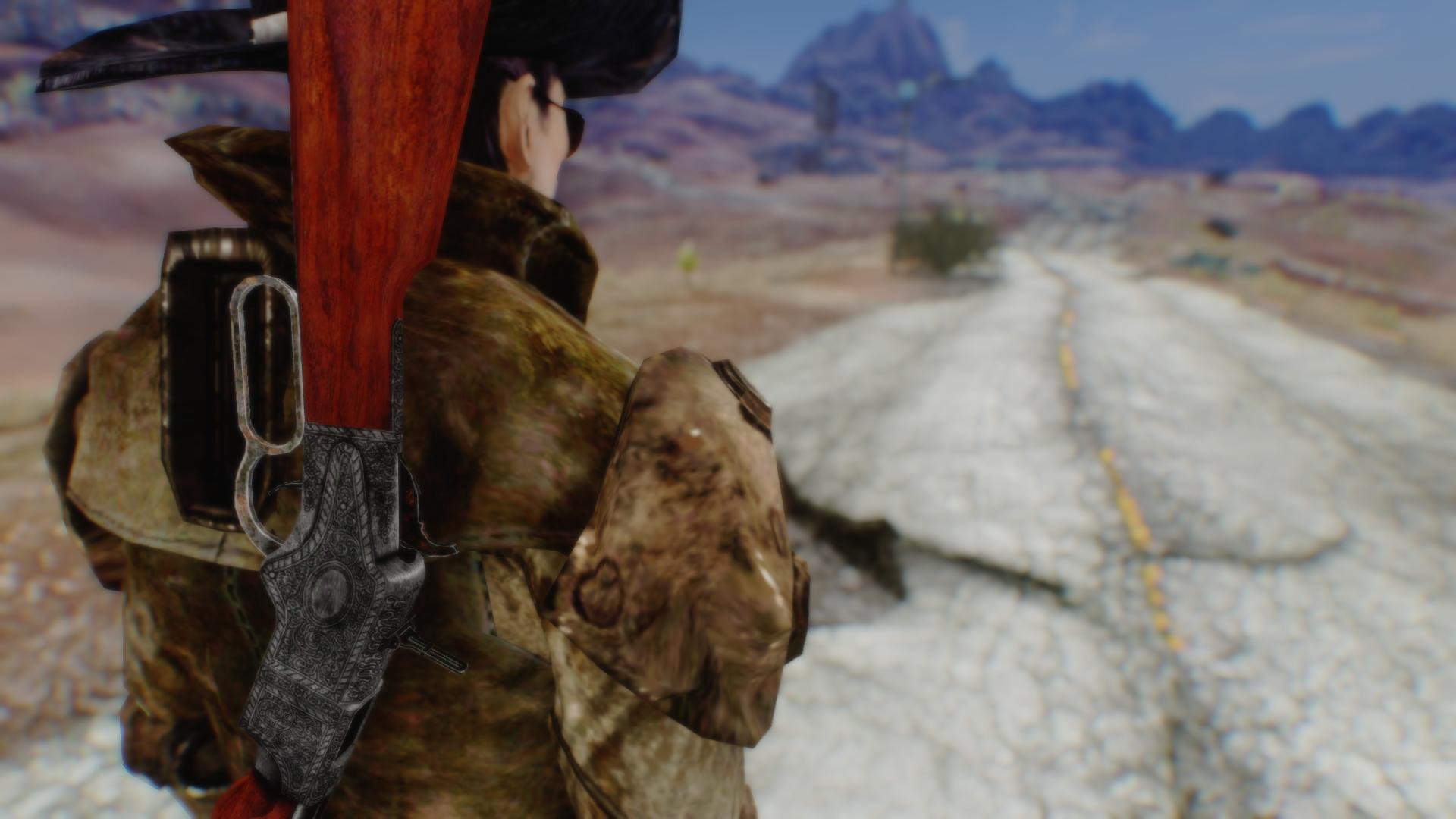The image depicts a lone figure standing on an ancient, cracked, and dilapidated concrete road that cuts through a barren desert landscape. The person, whose back is towards the viewer, is dressed in a vintage black or brown coat, possibly made from desert animal skins, and a distinctive cowboy hat that extends longer in the back. They have something attached to their back, resembling a mahogany rifle with intricate ironwork. The figure's attire includes puffy sleeves and khaki-colored clothing, giving them a rugged, old-western appearance. The scene is viewed from a perspective that makes it seem slightly blurry and surreal, much like a screenshot from a video game. The background features sparse, blurry brush and rocky mountains under a gray sky, evoking a sense of a post-apocalyptic, desolate environment, akin to the arid landscapes of southern New Mexico or Arizona. The cracked road, with visible yellow lines, further emphasizes the sense of abandonment and decay.